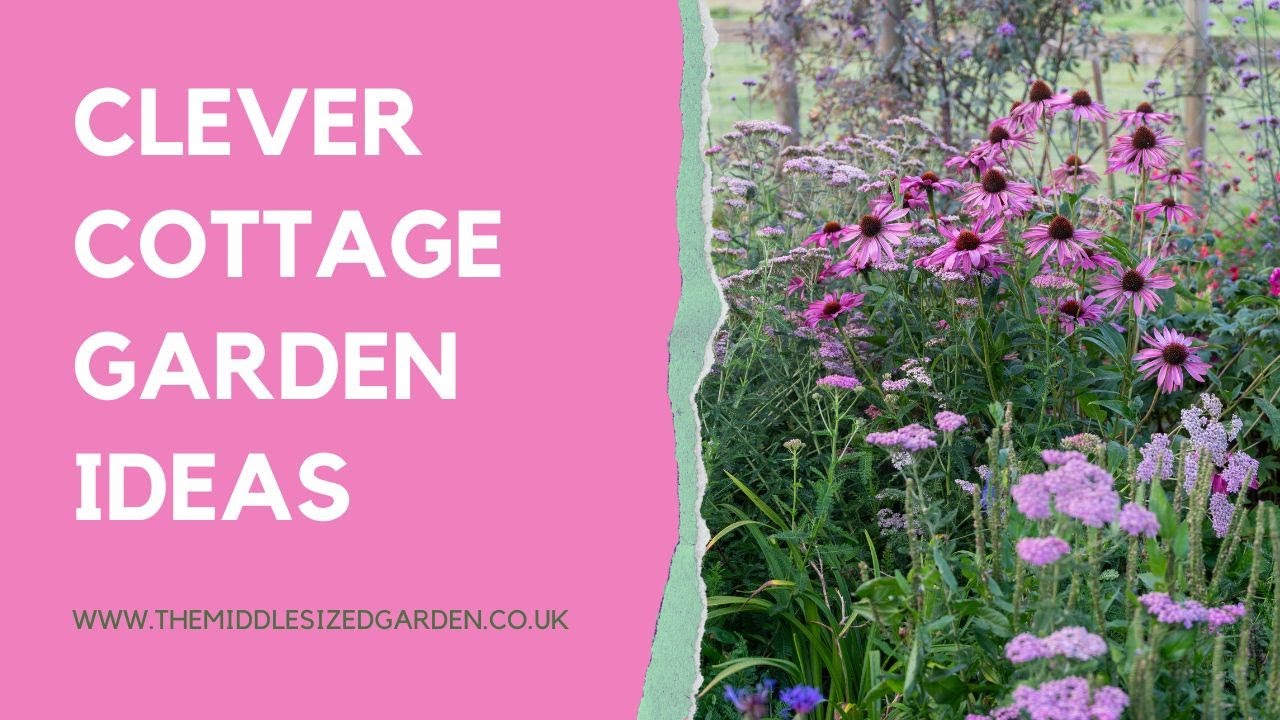The image is split into two main sections, with the left half featuring a pink background adorned with bold, all-capital white text that reads "Clever Cottage Garden Ideas." Below this, in a smaller, forest green font, also in all capitals, is the URL "www.themiddlesizedgarden.co.uk". This section has a greenish design element resembling a ripped page. The right half of the image showcases a lush garden scene filled with tall, blooming flowers. The flowers are predominantly pink with circular centers, gradually transitioning to purple as they reach the top. The background includes thin tree trunks and green grass, enhancing the natural outdoor setting with its vibrant and varied flora.